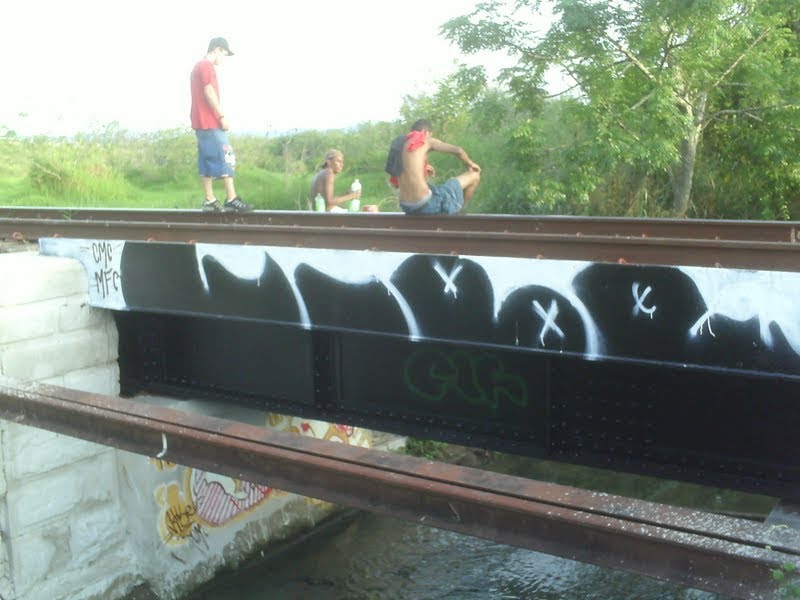The image captures a hot, sunny day with three boys on an old iron train bridge that spans over a creek. To the right of the image stretches a grassland meeting the sky, while to the left there are lush, green trees under a partly cloudy yet bright sky. The iron bridge runs horizontally across the frame, displaying rusted beams and adorned with graffiti—the black underside showcases white designs, X's, and letters "CMCMFC." Some yellow graffiti is scattered underneath, too. The bridge has weathered railroad tracks and a black base covered in graffiti, including on the banks near the water below.

On this bridge, three males are either sitting or standing. The boy on the right, distinguishable by his dark complexion, is wearing his baseball cap backward and clutching a big bottle of water in his right hand. He has a small bottle behind him. The boy in the middle is shirtless, with a black shirt slung over one shoulder and a red shirt draped over the other. He wears baggy pants exposing his underwear despite a visible belt and is seen scratching his bent knee with one hand while resting the other by his waist. The boy on the left, standing on the train tracks, wears a red t-shirt, baggy blue shorts ending just below his knees adorned with a pattern, and black sneakers or Crocs. He carefully navigates the rusty railroad tracks, adding dynamic movement to the otherwise relaxed scene.

The bridge's structure and surrounding nature create a picturesque juxtaposition, making it evident that the boys are taking a moment to relax and enjoy their youthful camaraderie against this industrial yet serene backdrop.